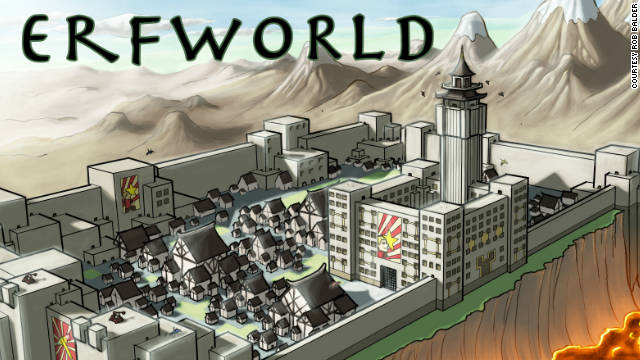This graphic illustration of a cartoon-style world, titled "Earthworld" at the top left corner (spelled E-R-F-W-O-R-L-D), depicts a vivid and intricate scene. The background reveals a range of brown mountains with snow-capped peaks under a blue and green sky dotted with clouds. To the left, additional hills of lighter tan shades enhance the landscape. 

Foregrounding the scene is a prominently featured city perched on the edge of a cliff, surrounded by a high gray concrete wall. This walled city centers around a towering main building or castle-like structure, characterized by a large turret and multiple windows. A prominent banner with red and white stripes, displaying a man’s face and a star, hangs from the main building, with two additional banners adorning other sections of the wall.

Inside the walled area, there is a courtyard populated with numerous white houses with brown A-frame roofs, resembling an old-fashioned village. The village includes similar-looking structures, with some houses clustering in the middle and a couple of businesses on one side. The cliff itself is brown and steep, dropping straight down to an ominous area of fiery red and yellow lava, giving the entire scene a dramatic and fantastical flair.